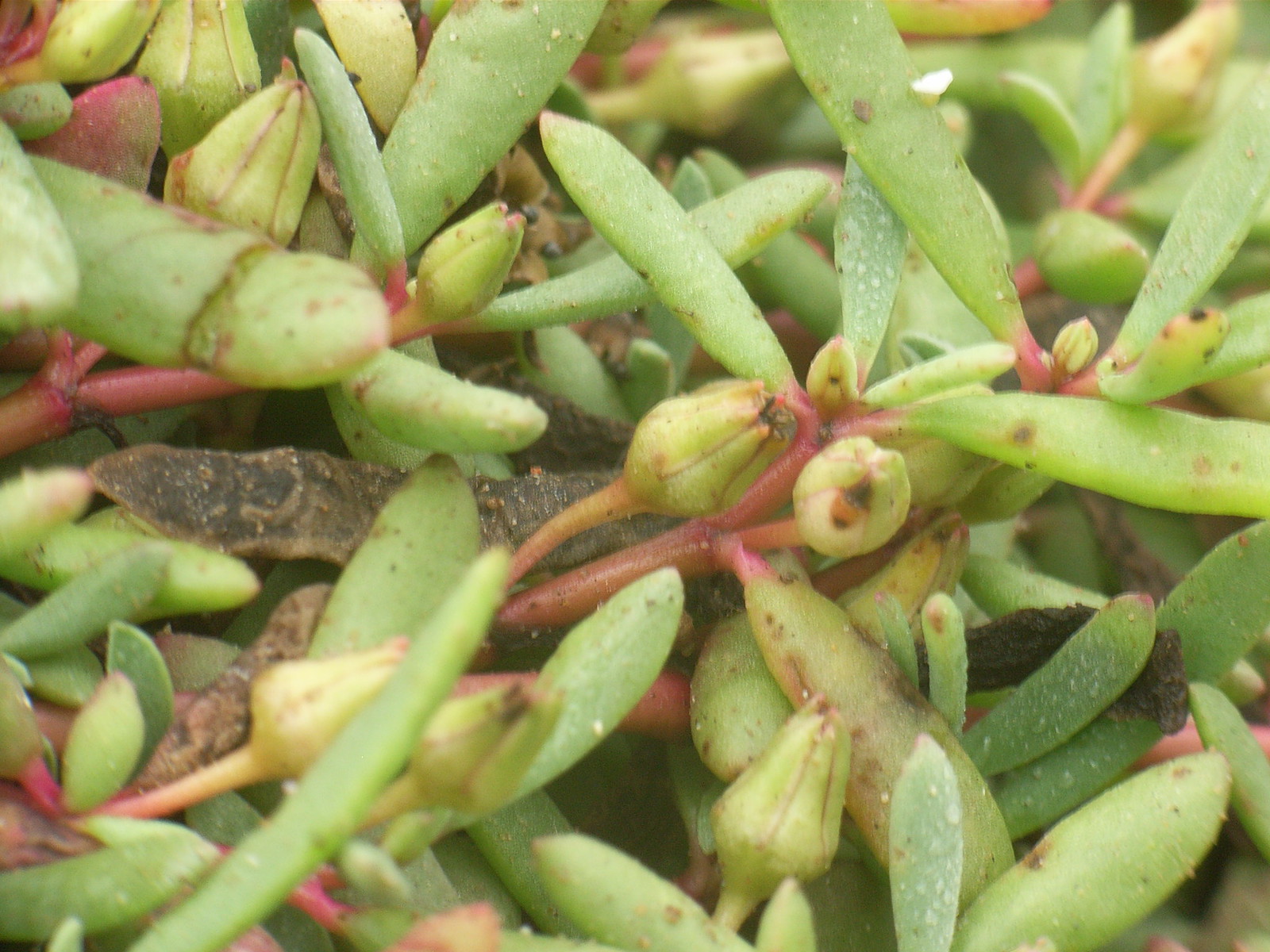This very close-up photograph depicts a succulent plant with puffy, snow pea-shaped leaves that are vibrant light green. The leaves have a somewhat thick texture, resembling smaller aloe vera leaves, and there are droplets of water on them, possibly dew or from recent watering. The plant features a central brown stem, with leaves connected by pink-tinged stems. Small, unbloomed flower buds are visible among the leaves. The lighting is good, suggesting the image was taken during the day, although the exact setting is unclear. The photograph appears slightly blurry and of low resolution, likely not captured with a professional camera. There's a single brown leaf present among the otherwise uniform green foliage. The image contains no text, people, date, or other identifying elements.